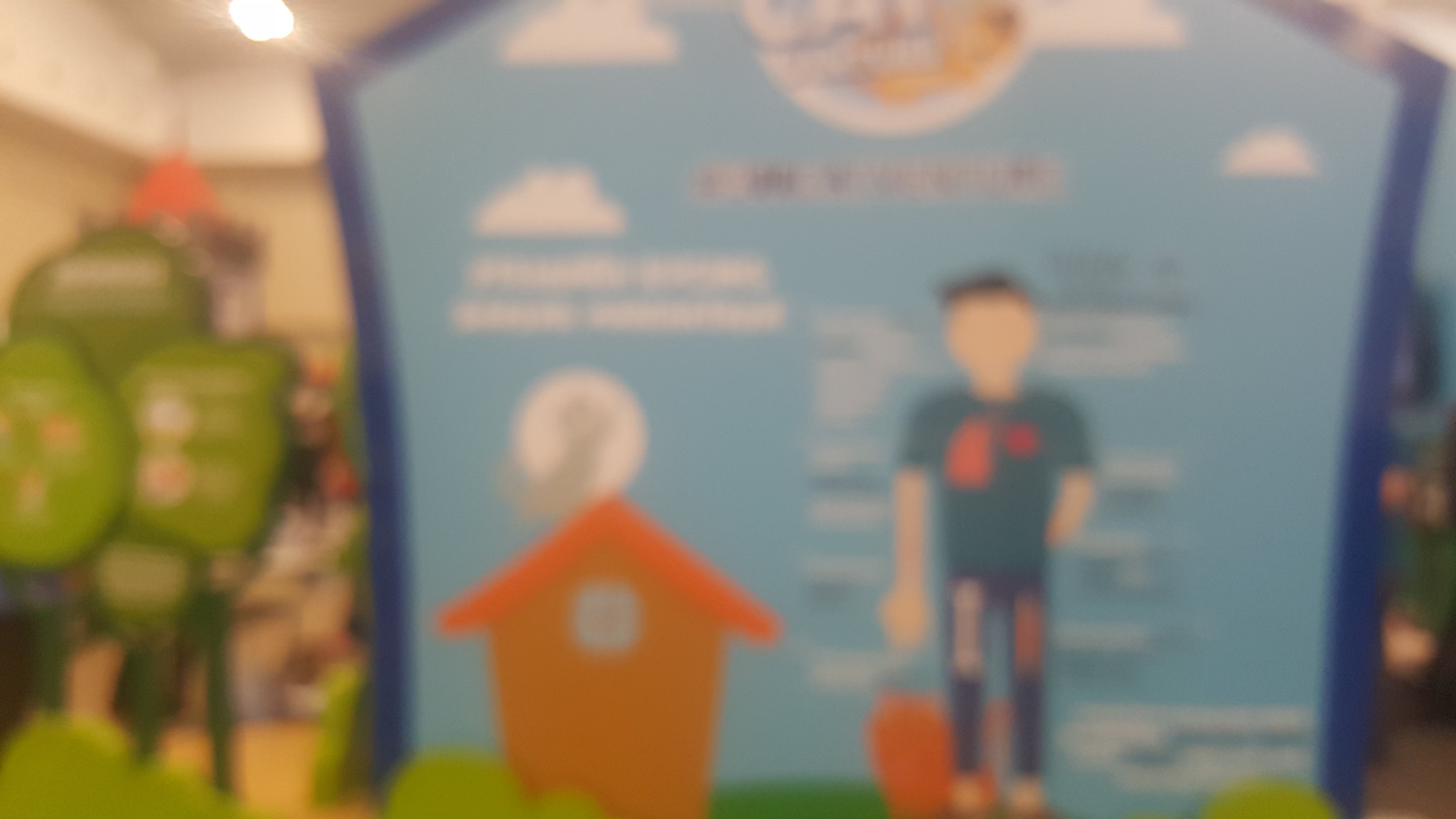The image shows a blurry, out-of-focus poster or sign. On the left side of the poster, there's a depiction of a tan ceiling with a white light, and below it, a series of four green circles with indistinct white details inside them, possibly representing another sign on a stand. Further to the left, there is a small orange structure resembling a doghouse or birdhouse with a brown wooden base, a gray hole in the center, and a V-shaped orange roof. On the right side of the image, there is a large blue outlined square with a light blue background, featuring a central figure of a young man with short black hair. He is wearing a greenish shirt with a decal on his chest that is too blurry to read, and dark blue pants. His shirt and pants have additional colors and patterns indicating anatomical features, such as possibly the heart, lungs, or bones. Surrounding the man, there are various blurred writings. The entire scene is set against a bright blue sky with fluffy clouds and a darker blue border, and the lower portion of the image shows patches of green grass. The setting appears to be an indoor space with brown walls and a white ceiling, where you can see one ceiling light.